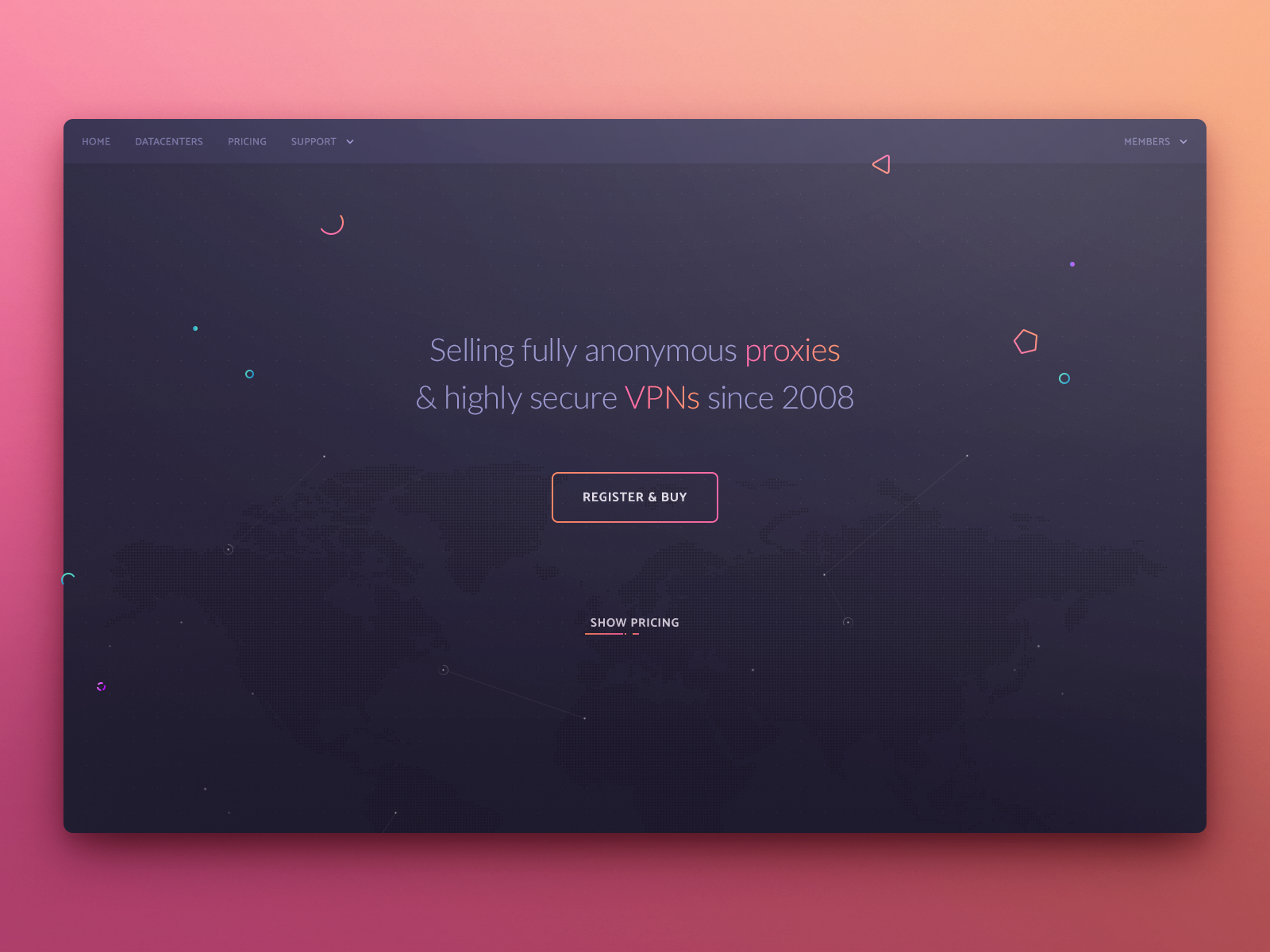The screen capture appears to be an advertisement, featuring a predominantly pink and orange-themed wallpaper background. The left side of the wallpaper is primarily orange, while the right side showcases various shades of pink, leaning towards a darker hue.

At the top of the screen, there's a large, black window with navigation options in a soft, purple-leaning blue font. The menu items are listed as "Home," "Data Centers," "Pricing," and "Support," with an adjacent pull-down menu. Another pull-down menu follows the label "Members."

The screen also features an assortment of icons, including an orange triangle, an orange semi-circle, an orange hexagon, and a blue circle. There are also some stray blue and purple markings scattered across the background.

In a combination of pink, orange, and purple-blue font, a highlighted slogan reads: "Selling fully anonymous proxies and highly secure VPNs since 2008." Below this, a white box with pink and orange borders includes the text "Register and Buy." Another white text box reads "Show Pricing," underlined with an orange line.

Overall, the image delivers a clear and concise message regarding the services offered, encapsulated in a visually striking and colorful design. There are no additional images or elements beyond what has been described.